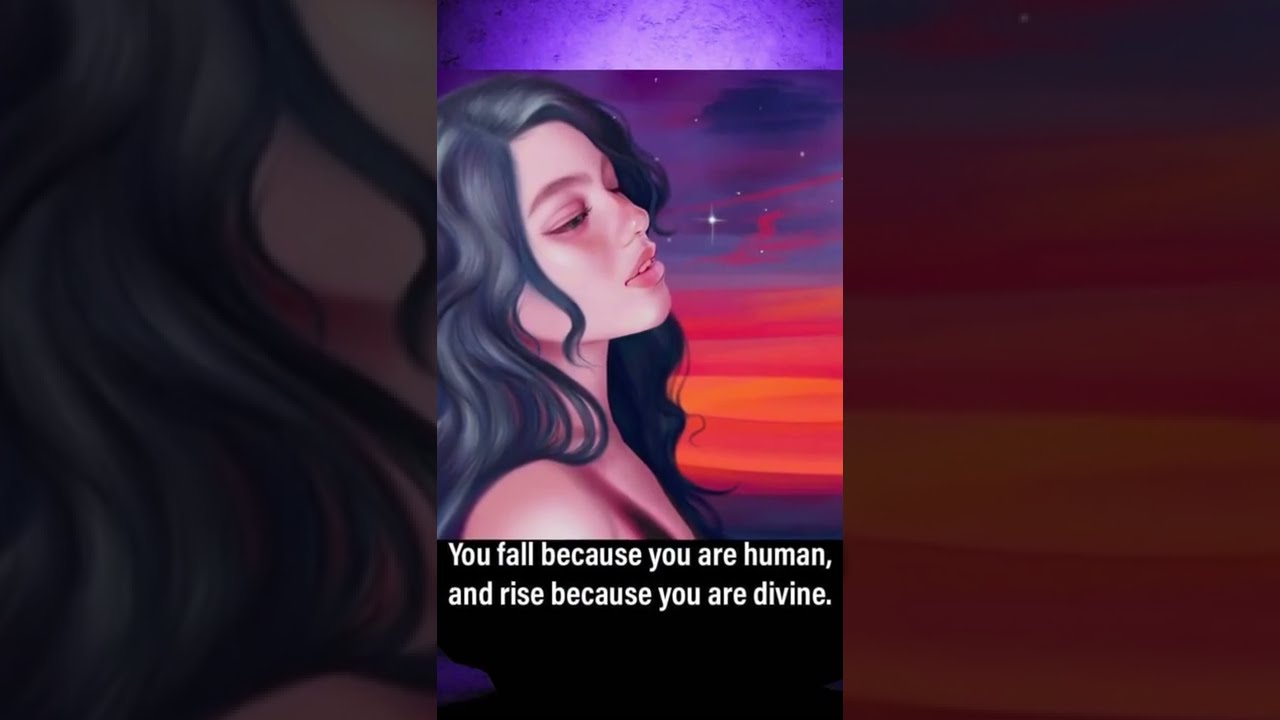The image is a digitally created, color illustration in a landscape orientation. At the center, there is a portrait of a young woman with long, flowing black hair cascading to the left. Her eyes are closed, and her head is tilted slightly upward, giving her an air of peaceful contemplation. She has soft shadowing on her face, with full lips softly parted, contributing to her overall serene beauty. 

Behind her, the sky transitions from a deep blue at the top, adorned with a single star, to vibrant orange and red hues at the bottom, suggesting a sunset or sunrise. The background is framed by a maroon square on one side and a design element on the other that complements the central image. Above this central portrait, there is a lavender gradient band that adds to the overall color harmony of the illustration.

Below the woman, the text reads, "You fall because you are human, and rise because you are divine." This inspirational quote is in white text, formatted in two centered lines against a black backdrop, enhancing its readability. The style of the entire piece is best described as illustrative fantasy, combining both realistic and whimsical elements that give the image a thoughtful and uplifting atmosphere.